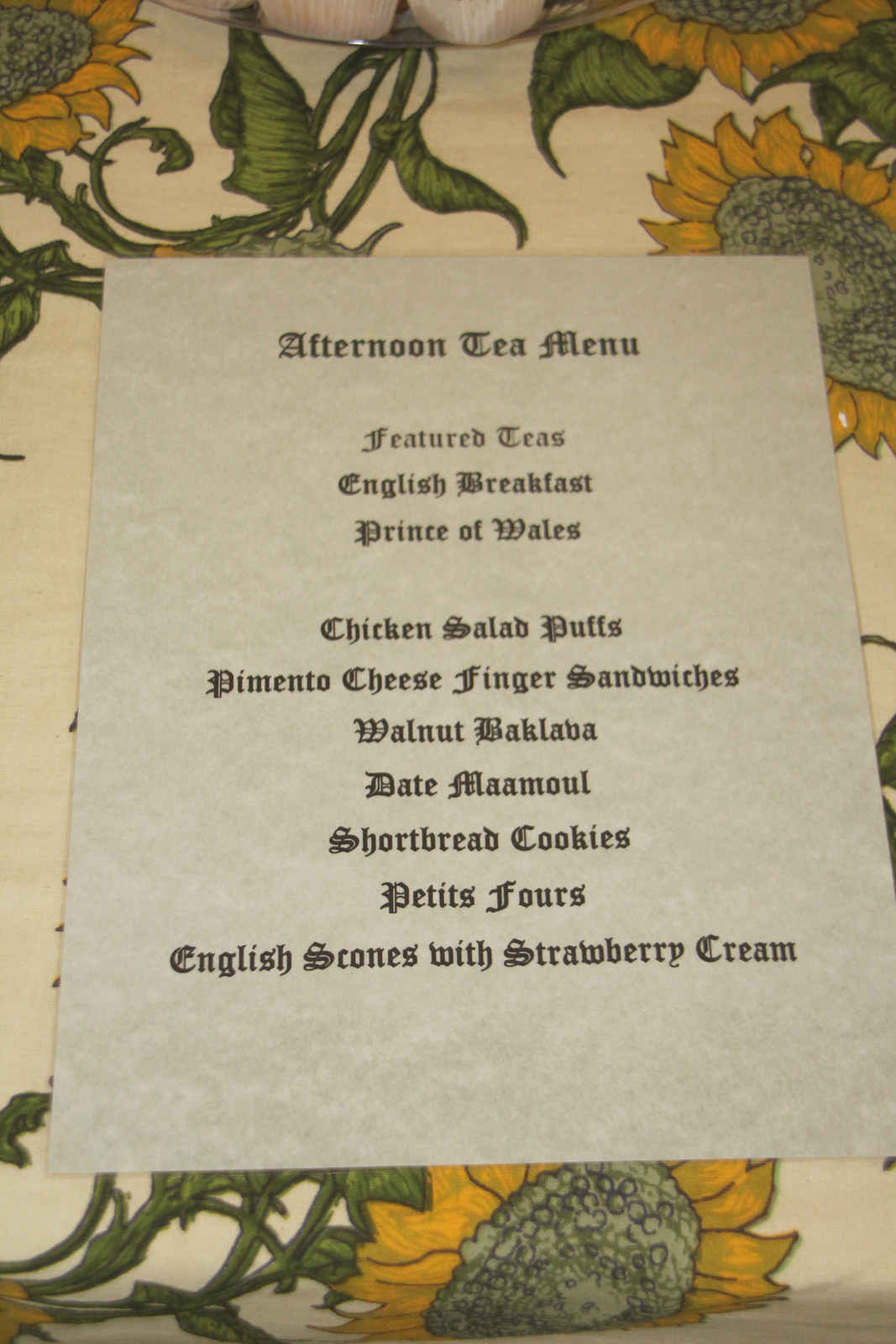The image depicts a laminated afternoon tea menu placed on a table covered with a detailed cream-colored tablecloth adorned with large, vibrant yellow sunflowers with black centers and green stems and leaves. The menu itself features an old-fashioned, almost medieval black font and lists the offerings: "Afternoon Tea Menu," "Featured Teas - English Breakfast, Prince of Wales," followed by "Chicken Salad Puffs, Pimento Cheese Finger Sandwiches, Walnut Baklava, Date Mamoul, Shortbread Cookies, Petit Fours, and English Scones with Strawberry Cream." Above the menu, a clear tray displaying what appears to be white cupcake holders is visible, adding to the elegant and inviting ambiance.